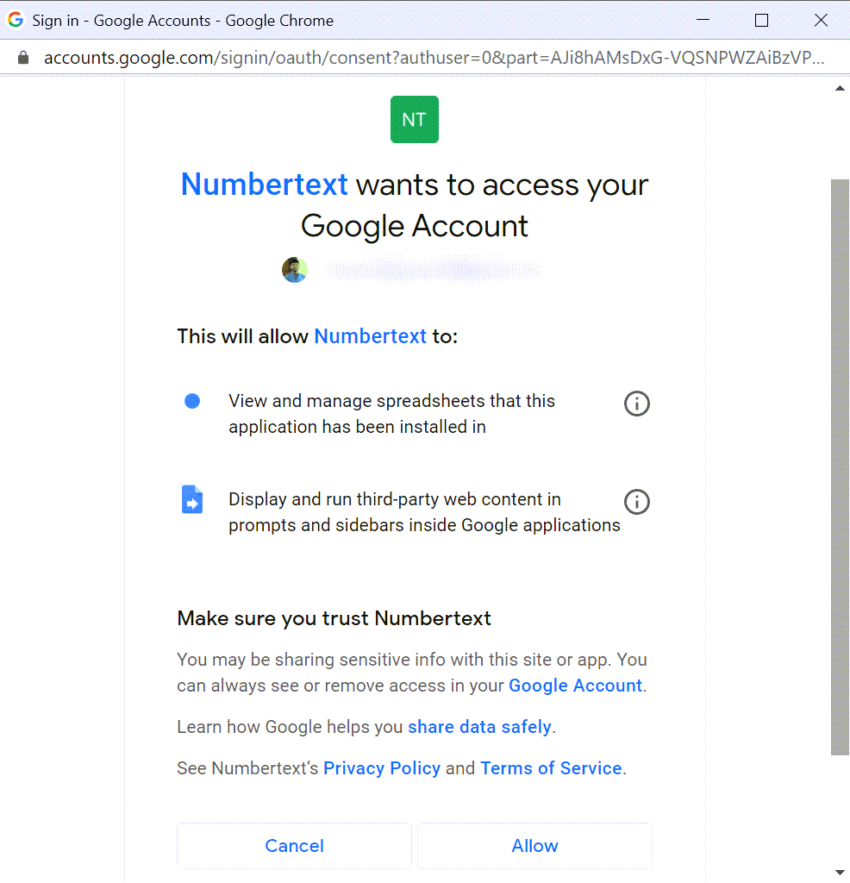A detailed description of a screenshot showing a Google sign-in or authorization page:

---

The screenshot features a typical Google sign-in or authorization interface. At the very top of the window, in the title bar, it reads "Sign in to Google Accounts - Google Chrome." Directly below the title bar, the URL bar is visible, though its contents aren't specified.

Centrally positioned at the top of the main page, there is a compact, square icon with the letters "NT" inside. Directly beneath this icon, a message in black and blue text states: "Number Text wants to access your Google Account." The words "Number Text" are specifically highlighted in blue, while the rest of the text remains black, ensuring clarity and prominence.

Below this introductory section, a circular profile picture is displayed alongside a blurred-out Google account name, maintaining user privacy. Under the profile picture, a brief statement clarifies the app's permissions: "This will allow Number Text to." Further down, there are detailed bullet points describing the extent of the permissions:

1. View and manage the spreadsheets that this application has been installed in.
2. Display and run third-party web content, prompts, and sidebars inside Google applications.

Each permission has a corresponding informational icon, represented by an eye inside a circle, positioned to the right, allowing users to obtain more details if needed.

Proceeding further, a concise reminder advises users, "Make sure to trust Number Text." The page concludes with a duo of action-taking options at the bottom. Two buttons, "Cancel" and "Allow," are distinctly outlined; the "Cancel" button features blue text, while both buttons are encased in a thin gray border, ensuring they stand out for user interaction.

---

This detailed description ensures a clear understanding of the visual and textual elements present in the Google authorization page screenshot.